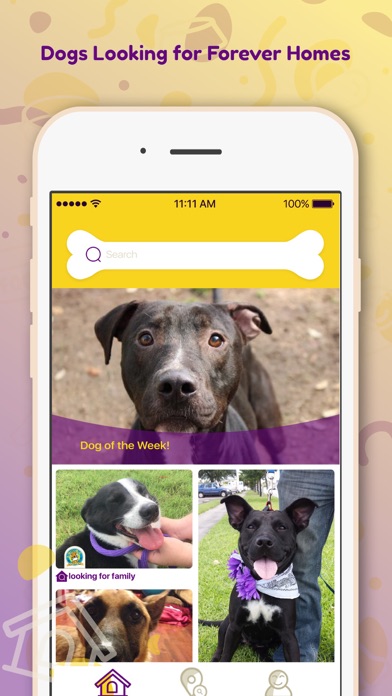This vibrant screenshot captures a dog adoption website or app interface, designed to help dogs find their forever homes. The background features a vivid gradient transitioning from yellow to purple, adding a lively and engaging atmosphere. Displayed prominently on the screen is a digitally generated image of a smartphone resembling an iPhone, with the clock displaying 11:11 AM in the middle.

At the top of the interface, there's a whimsical search bar shaped like a dog bone, encased in a yellow box, complete with a magnifying glass icon and the word "Search" within it. Showcased at the top of the screen is a highlighted image labeled "Dog of the Week," framed by a purple, half-circle banner with the label in bold yellow text just below it.

Beneath the featured dog, three smaller photos present additional dogs, each accompanied by the label "Looking for Family," indicating their readiness for adoption. The bottom section of the screen hosts a navigation bar featuring three icons: a house representing the home page, a map pin for location services, and an avatar symbolizing user profiles.

Overlaying the entire screen, subtle doodles of houses watermarked in the background further emphasize the theme of finding permanent homes for these adorable pets.